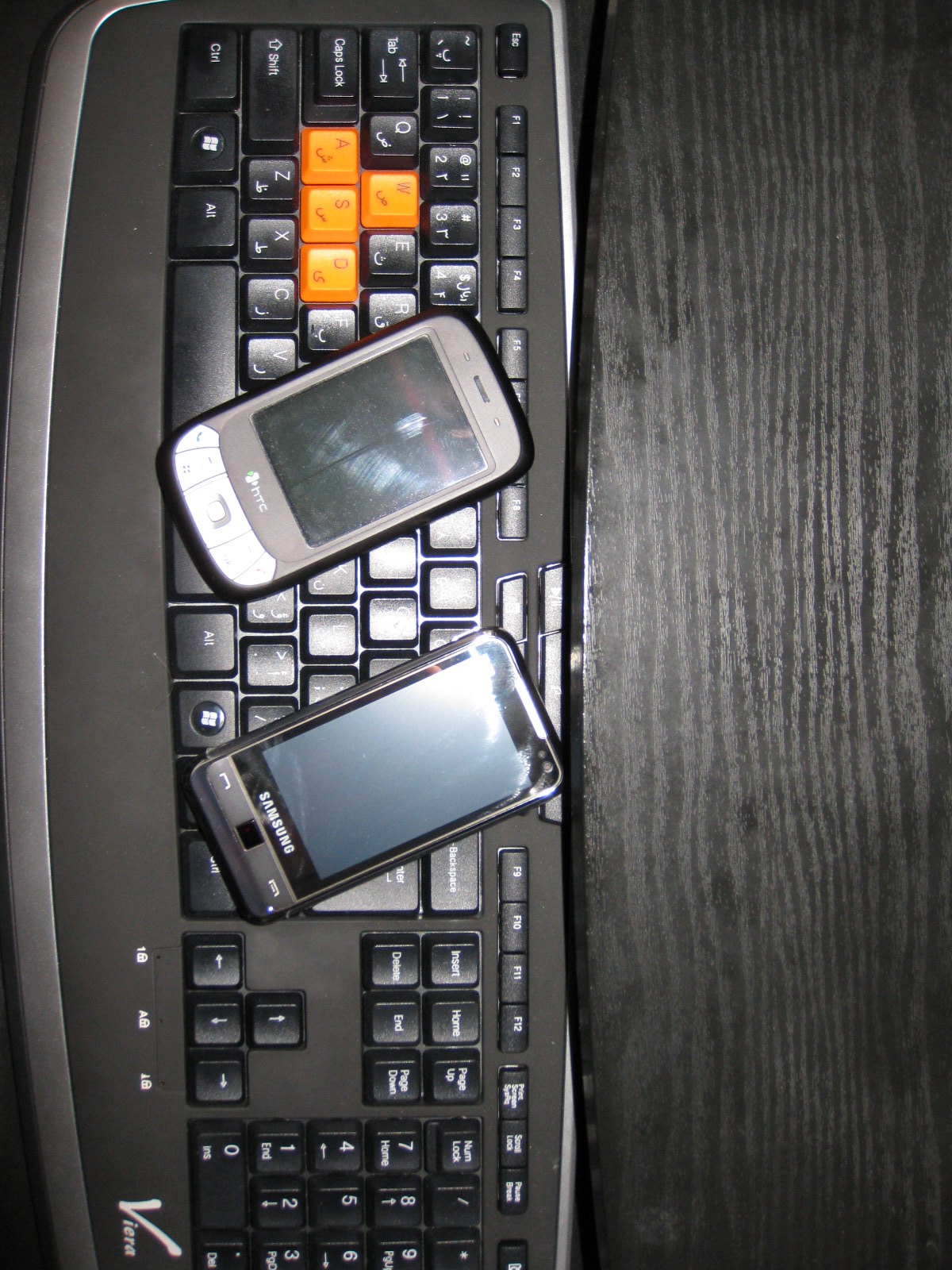The photo captures a close-up shot of a computer keyboard on a simulated wood grain desk, which appears to be either a very dark wood or charcoal gray color. The keyboard is marked with the brand "Viera" and is predominantly black with white lettering, except for the orange WASD keys which stand out, suggesting either a custom modification or a specific design feature. Situated across a section of the keyboard are two early-model smartphones: one from HTC with a small touchscreen, and an older Samsung model featuring both a touchscreen and physical hang up/pick up buttons. The image has a somewhat blurred quality and crops some portions, focusing mainly on the arrangement of the phones and keyboard.